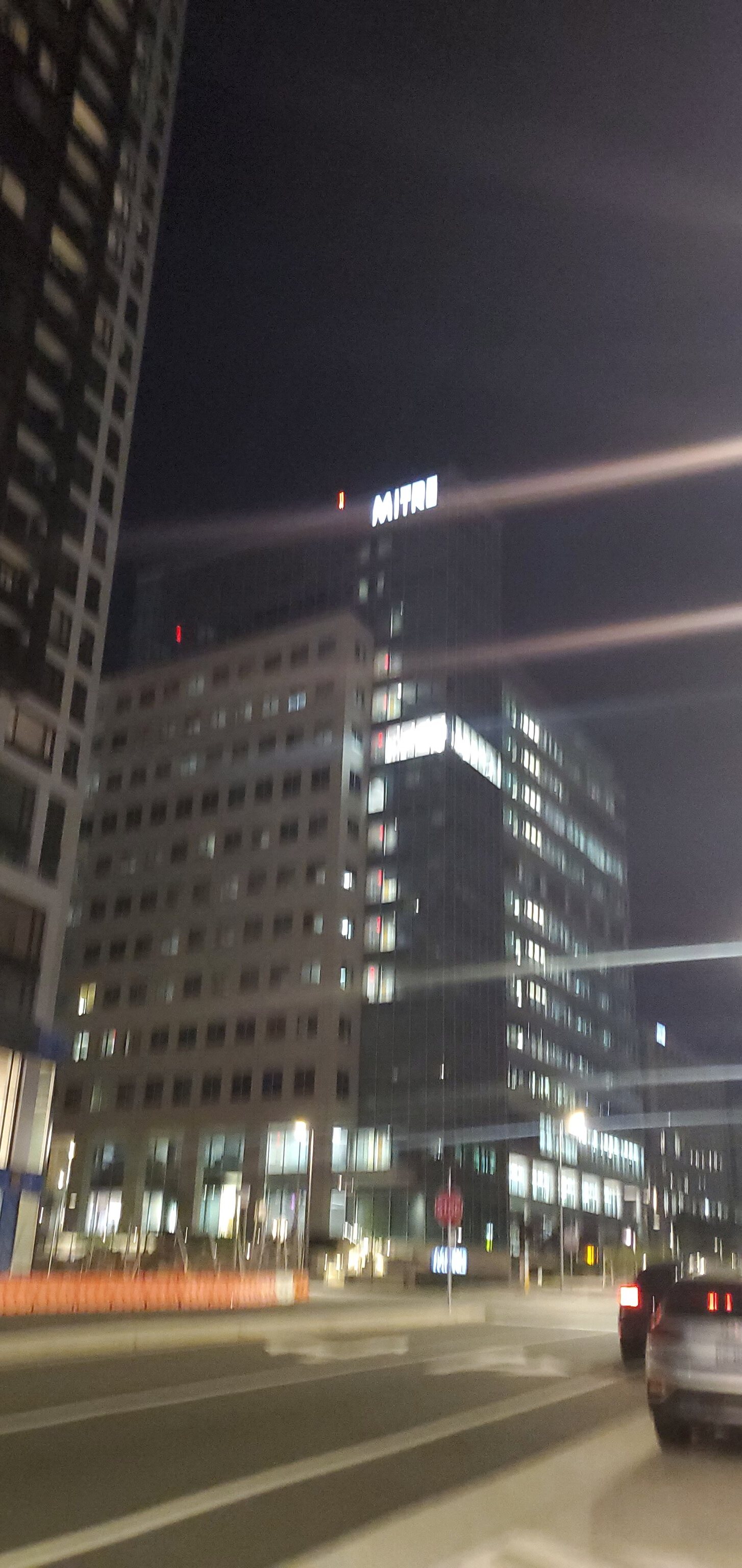The photograph captures a bustling downtown cityscape at nighttime, presenting a vivid and detailed depiction of urban life. In the foreground, a dark gray road with distinct white street markings runs through the scene. A silver vehicle and a black vehicle are prominently visible on this road. On the opposite side of the street stands an orange barrier.

A red stop sign with bold white lettering can be seen in the background, adding a touch of vibrant color to the scene. The city skyline fills the backdrop with a mix of silver and black skyscrapers adorned with numerous windows. Soft white lights shine from several windows, creating a warm contrast against the dark night.

Dominating the center of the image is a tall black skyscraper. At its peak, an illuminated sign, though too blurry to decipher, glows with white light. An orange light is also visible atop this building, adding to the city's nocturnal ambiance.

A striking visual feature of the photograph is a streaking effect that cuts across the middle of the image, suggestive of fast-moving lights or extended exposure capturing the dynamism of city life.